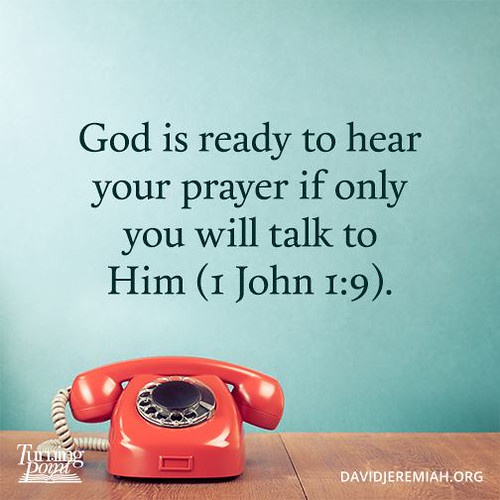The image is a square, color photograph with a blend of typography and graphic design, presenting a religious advertisement. The scene is set against a light blue background with a green tint. Dominating the bottom eighth of the image is a beige wooden tabletop. Positioned on the bottom left of the table is an old-fashioned, rotary dial phone, colored in a bold red-orange with a tan cord, contrasted by black ring dials.

Above and centered on the background is a navy blue script message that reads: "God is ready to hear your prayer, if only you will talk to him. (1 John 1:9)." 

On the lower left corner of the image, the brand "Turning Point" appears in small white print, while the lower right corner features the web address "DavidJeremiah.org" in the same white font. The design, suggestive of realism combined with graphic elements, serves to hint that reaching out in prayer is as straightforward as making a phone call.